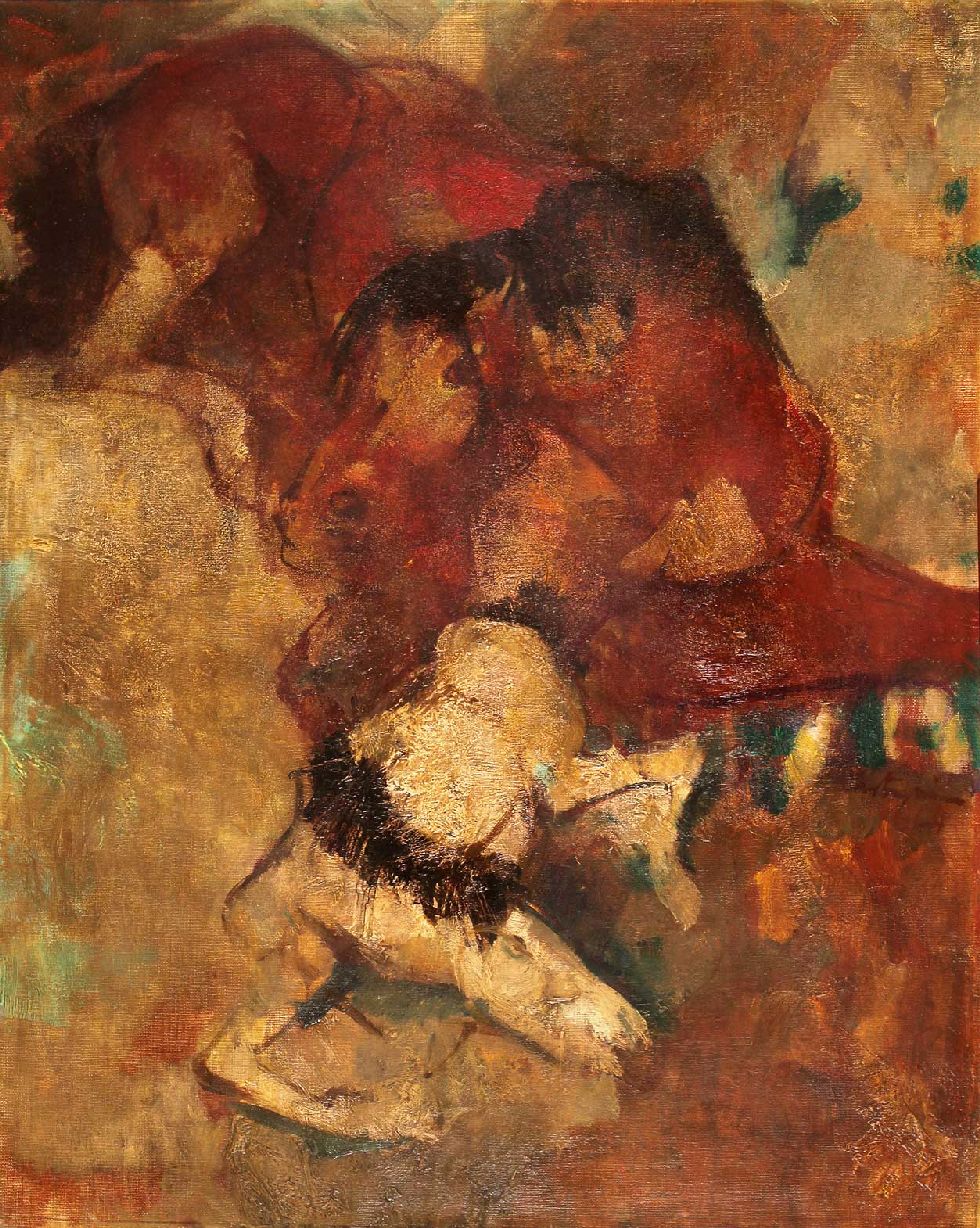The image is an abstract painting, rich with warm and earthy tones like red, orange, brown, tan, beige, and accents of green, white, black, blue, and burgundy. Dominated by the color red, this complex and layered artwork seems to play with the viewer's perception, akin to a Rorschach test. Several indistinguishable objects are intertwined, creating a collage that is open to interpretation. Central to the painting is the suggestion of a horse, possibly in a seated or reclining position, extending from the upper left corner into the center, with its black mane prominently visible. Below or intertwined with this figure, one might discern the form of a smaller horse or foal, appearing to struggle as if newly born. Amidst the chaotic and mashed-together elements, hints of an animal's eye, whiskers, and nose can also be detected centrally, adding to the painting's mysterious and almost cave-like aesthetic. The medium appears to be either oil or acrylic, contributing to the textured, layered style of the artwork.